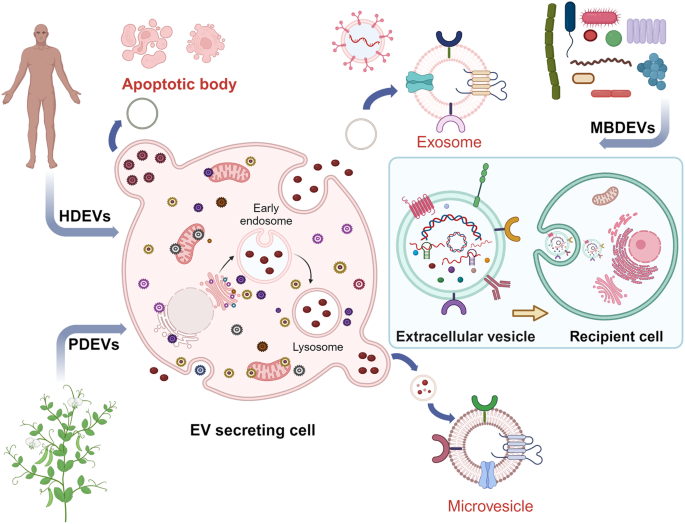The image is a detailed scientific diagram likely intended for an anatomy or medical textbook, illustrating the process of extracellular vesicle (EV) secretion and their roles in cancer and tumor biology. In the top left corner, there is a human figure emitting HDEVs while in the bottom left, a plant is shown emitting PDEVs. Both types of vesicles are directed by arrows toward a large, prominently featured EV-secreting cell depicted in pale pink hues. This cell highlights key components such as lysosomes and early endosomes, and various internal structures resembling caterpillars and chocolate chip cookies or doughnuts. Additionally, there are smaller diagrams including exosomes, visualized as pink doughnuts with colored patterns. The infographic uses a color palette of pale pinks, lilacs, greens, pale blues, and mauves to distinctively mark different parts and processes, illustrating how the EV-secreting cell processes and distributes ingested compounds throughout the body.